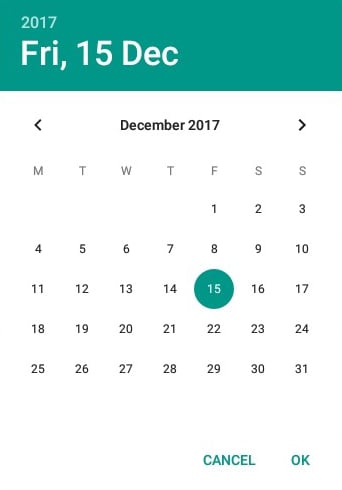This image is a screen capture of a digital calendar page displaying December 2017. At the top, there is a large, teal-colored box featuring the year "2017" in teal font. Below this, the date "Fry, 15 DEC" is displayed in bold white font. Directly beneath that, there are back and forward navigation arrows in black, with "December 2017" written between them, also in black. The text in this section appears slightly pixelated and grainy.

The days of the week—Monday through Sunday—are listed in gray, and the calendar layout for December starts on a Friday. Each day of the month is marked with numbers in a blackish-gray font, except for the 15th, which is highlighted with a teal circle and the number displayed in white, indicating it is the selected date.

At the bottom of the image, two teal-colored buttons read "Cancel" and "OK." The image is simplistic with no additional objects or images. The "DEC" part of the date is blurry but still legible, giving the entire calendar a slightly wavy, pixelated appearance.